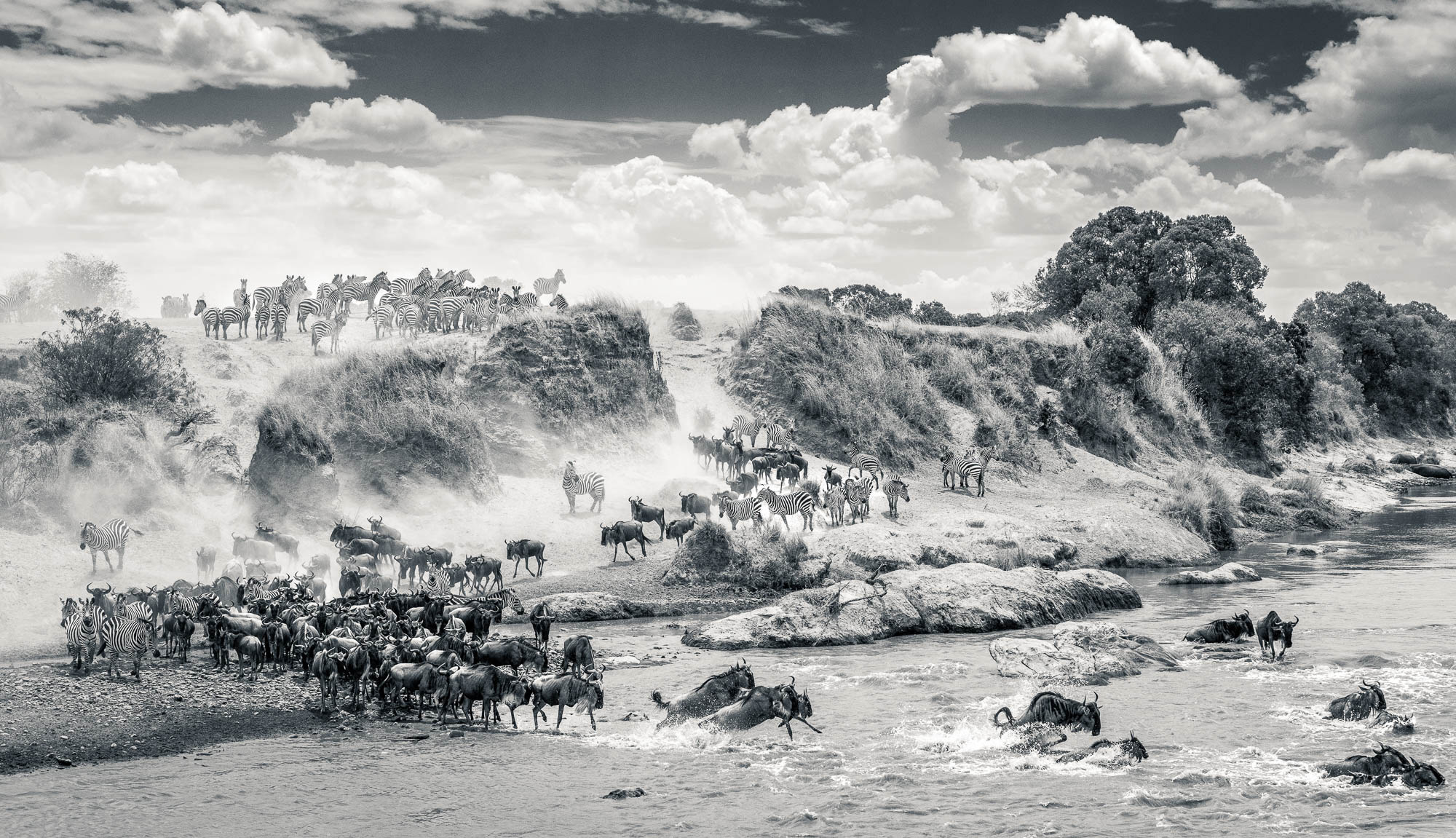This detailed black and white, high dynamic range photograph captures a bustling scene in Africa. The landscape features dusty, grassy, and rocky hills scattered with trees. Prominent in the foreground is a river, with a large number of water buffalo either crossing or preparing to cross, their behavior suggesting urgency or danger. To the left, a substantial herd of zebras, possibly up to a hundred, congregate on the hillside and at the riverside, some venturing into the water. The sky above is filled with large, puffy white clouds, adding depth and contrast to the image. The scene is meticulously detailed, with the lifelike representation of the animals and landscape making it difficult to discern whether it's an artistic creation or a real photograph.